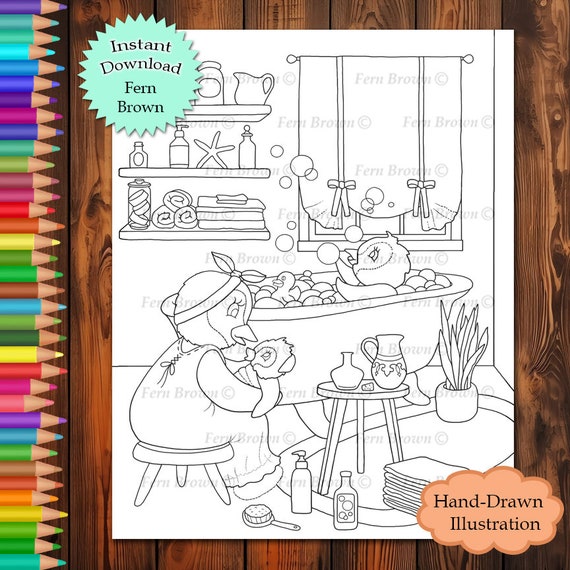This is a black and white line drawing printed as a coloring page on a single sheet of white paper, designed to be colored with a full set of colored pencils. The background features heavily grained and heavily stained brown wood. A zigzag starburst design in the top left corner, with a mint green background, bears the text "instant download Fern Brown" in brown and black lettering. In the bottom right corner, a tan cloud states "hand drawn illustration" in dark brown lettering. Along the left edge of the sheet is an array of finely sharpened colored pencils showing the complete spectrum of the rainbow.

The central image depicts a detailed bathroom scene with a bear bathing in a bubble-filled tub. To the left of the tub, a duck sits on a stool holding a teddy bear. The floor displays various bottles, towels, a potted plant, and another stool with pictures on it. Behind the tub, a window with drawn curtains, each adorned with striped pieces and bows at the bottom, provides a backdrop. In the top left corner, three wall-mounted shelves hold an array of pictures, bottles, a starfish, some rolled towels, an apothecary jar, and other bath items, completing the intricate display ready for coloring.